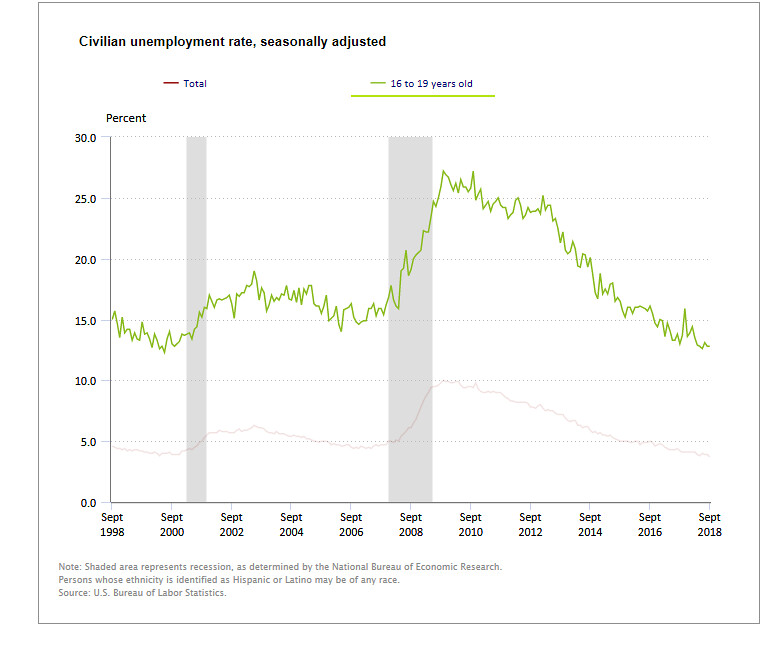The image is a detailed line graph depicting the civilian unemployment rate, seasonally adjusted, from September 1998 to September 2018, set against a white background. At the top, "Civilian Unemployment Rate, Seasonally Adjusted" is written in black text. There is a legend indicating a green line for unemployment rates among individuals aged 16 to 19 years old and a red line for the total population. 

On the left vertical axis, the graph is marked with percentages ranging from 0% at the bottom to 30% at the top. Along the bottom horizontal axis, multiple data points are labeled by year at two-year intervals from September 1998 to September 2018.

The green line, representing the 16 to 19-year-old age group, starts at approximately 15% in 1998. It remains relatively steady until 2007, where it spikes significantly, peaking around 27% during the 2008-2009 recession before decreasing to about 11% by 2018. The red line, denoting the total civilian unemployment rate, starts at roughly 5% in 1998, displays minor fluctuations until 2007, then shows a notable rise during the same recession period before stabilizing back to around 5% by 2018.

Gray shaded bars highlight recession periods, as determined by the National Bureau of Economic Research, specifically around 2001 and 2008-2009. Additional notes in the lower left corner explain that individuals identified as Hispanic or Latino may be of any race. The source of the data is cited as the US Bureau of Labor Statistics.